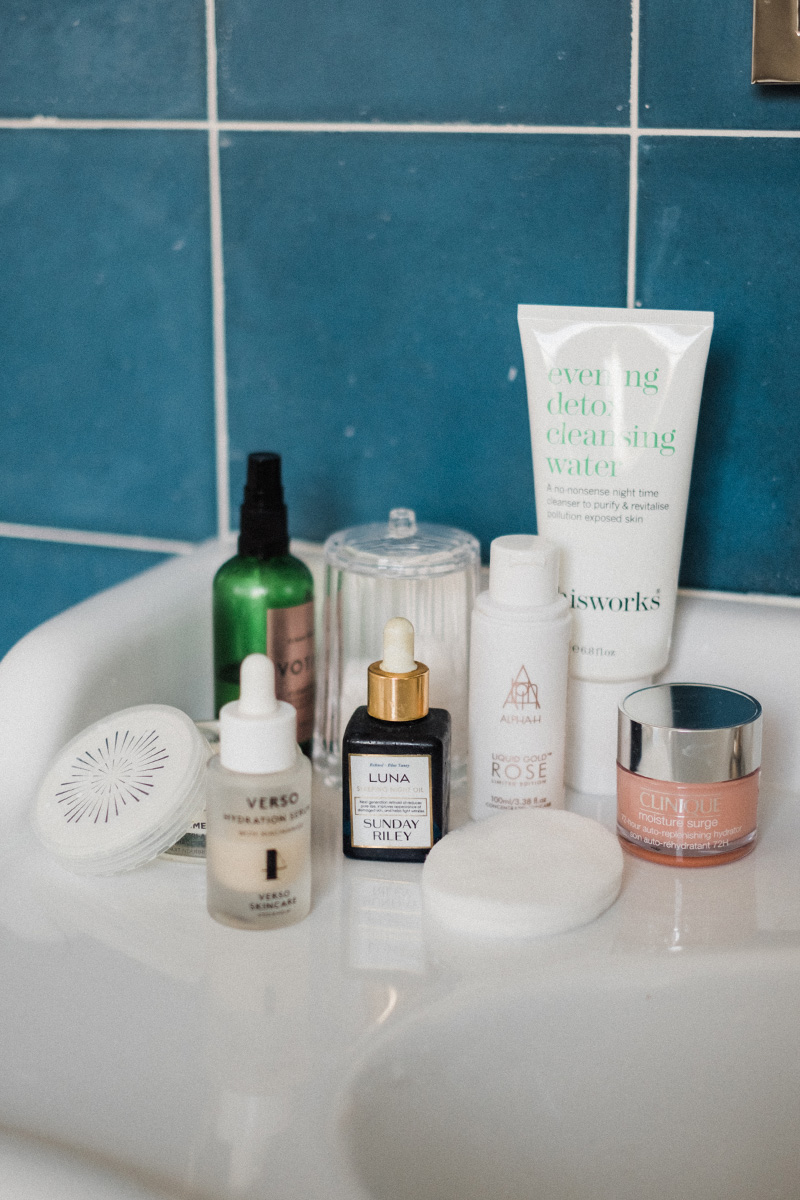A close-up image of a pristine, all-white kitchen sink showcases a variety of personal care and cleaning products neatly positioned on the right corner. The backdrop consists of light blue tiles with white grout, contributing to a clean and serene aesthetic. Among the assorted products, distinctive labels such as Luna, Verso, and Riseworks are visible, indicating their purpose as either cleaning agents or lotions. A notably smaller bottle of Clinique Moisture Surge stands out with its peach color. There is also a bar of soap, alongside several disc-shaped items that closely resemble soap bars, although their exact nature is unclear. A green bottle is placed towards the back, while a darker bottle is prominently situated in the front. In total, there are approximately seven bottles arranged on the sink. The glossy porcelain surface of the sink reflects some of the bottles, adding depth to the composition. The upper right corner of the image subtly reveals the edge of a mirror, contributing additional reflections and glare to the scene. A few tiny white specks can be seen on the blue tiled wall, suggesting minor imperfections or dirt.